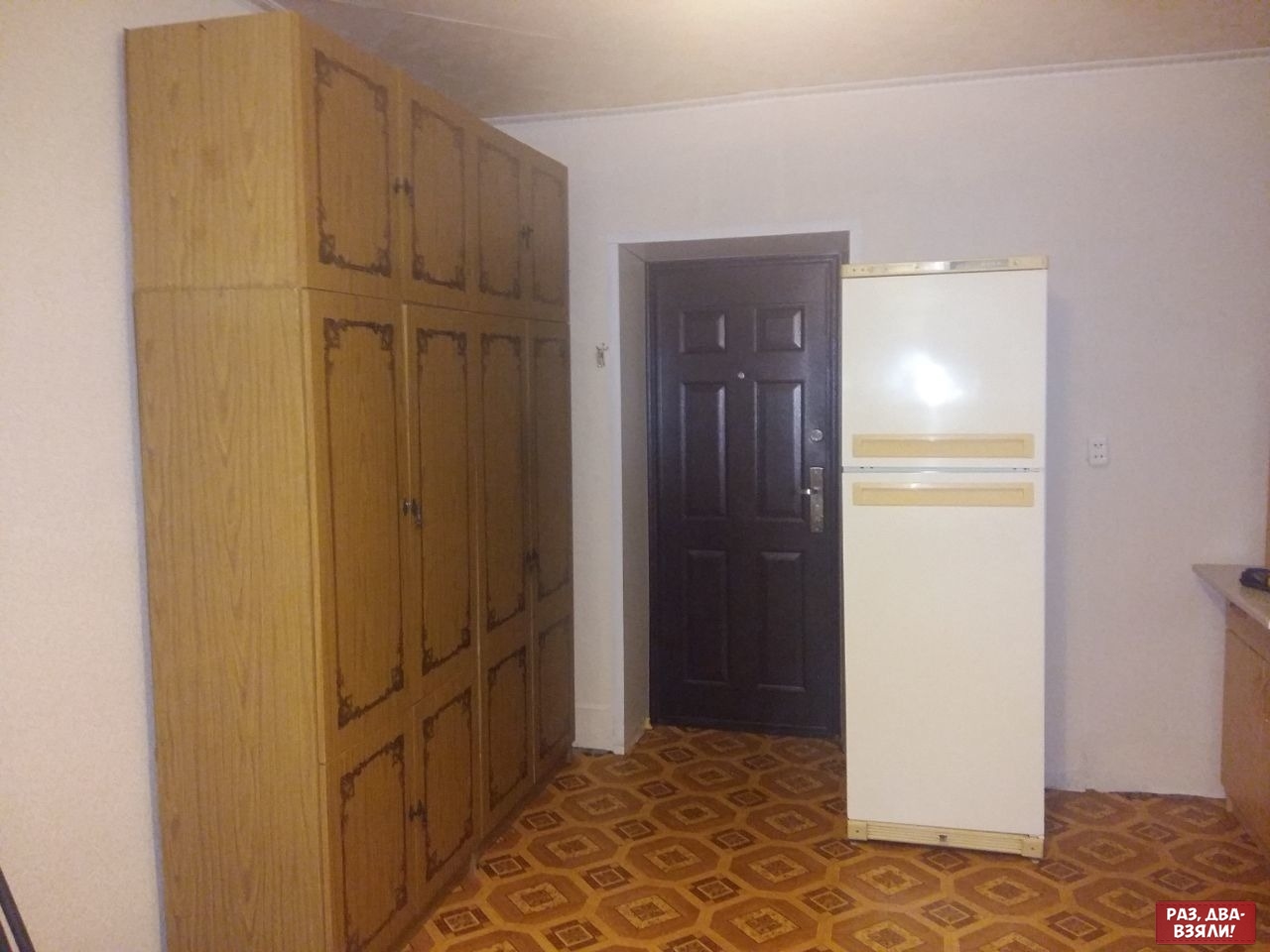This is a color photograph capturing a modest kitchen interior, highlighting various elements with a focus on a black external door at its center. The door, seemingly crafted from heavy wood with decorative panels and equipped with a silver deadbolt and a peephole, directly leads into the kitchen. To the left of the door, there is an expansive storage unit comprising a series of closed, brown, wood-grain cabinets with metal handles. The cabinet configuration includes tall double door sections with smaller compartments above, providing ample storage space. 

On the right side of the door is a slender, outdated white refrigerator, characterized by its top freezer and bottom refrigerator design, with some orange rectangles near the crease and a subtle reflection on the freezer door hinting at its aged texture. Adjacent to the refrigerator, partly visible, is a countertop made of stone or laminate, supported by wood cabinets below. 

The flooring is covered with old-fashioned linoleum tiles featuring a pattern in shades of orange and brown, forming geometric shapes. The surrounding walls are painted white, contributing to the kitchen's bright ambiance despite the photograph's low quality, which suggests a slightly blurred or puffy effect due to a possible dirty lens. An electrical outlet can be spotted near the refrigerator, and to the far right, the image captures a glimpse of additional cabinet space and a countertop, possibly hosting a sink. Notably, there is also some Russian writing located at the bottom right corner of the image. Overall, this kitchen appears functional yet dated, reflecting a blend of practical storage solutions and traditional design elements.